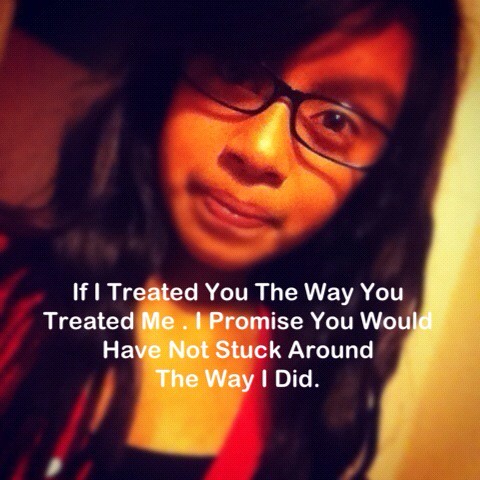The image features a girl with slightly wavy, long black hair and rectangular black plastic-framed glasses. She has dark brown eyes and a side bang partially covering one eye. Her facial expression is neutral, with slightly pursed lips, and she is looking directly at the camera. She appears to be wearing a black tank top and possibly a red scarf or shirt over it. The image has a reddish-yellow filter, giving it an orange and yellow hue, which highlights her face and chest in warm tones. Overlaying the image, there is white text, positioned over her chest, that reads: "If I treated you the way you treated me, I promise you would not have stuck around the way I did," with each word's initial letter capitalized. The background transitions from yellow on the right to orange on the left, further contributing to the filtered effect of the photo.